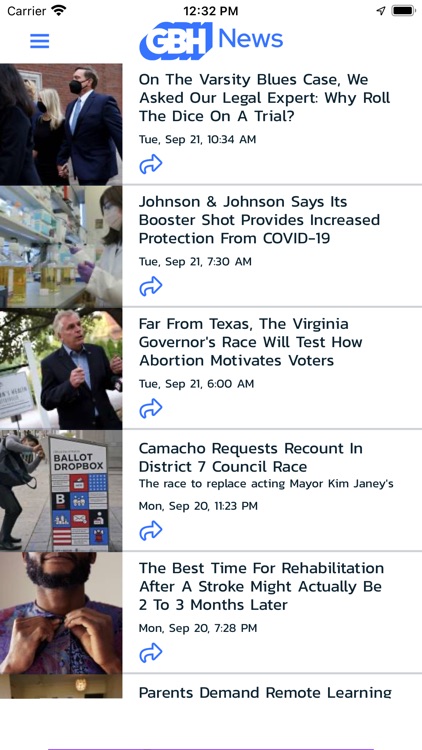This image, set against a white background, appears to be a screenshot of a tablet displaying a news website. At the top left, the status bar shows the carrier name and the Wi-Fi icon centered, indicating a connected status, along with the current time of 12:32 PM. The upper right corner displays a fully charged battery icon. 

In the main content area, there is a header with "GBH News" in blue text against a blue, three-dimensional background. To the left of the text is the menu icon featuring three horizontal lines.

The leading headline reads: "In the Varsity Blues Case, We Asked Our Legal Expert: Why Roll the Dice on a Trial?" dated Tuesday, September 21st at 10:34 AM. Below this headline, an image shows several individuals in a courtroom, all wearing black face masks. 

Subsequently, another headline states: "Johnson & Johnson Says Its Booster Shot Provides Increased Protection from COVID-19," dated Tuesday, September 21st at 6:00 AM.

The final article at the bottom of the screen discusses stroke rehabilitation: "The Best Time for Rehabilitation After a Stroke Might Actually Be Two to Three Months Later," dated Monday, September 20th at 7:28 PM.